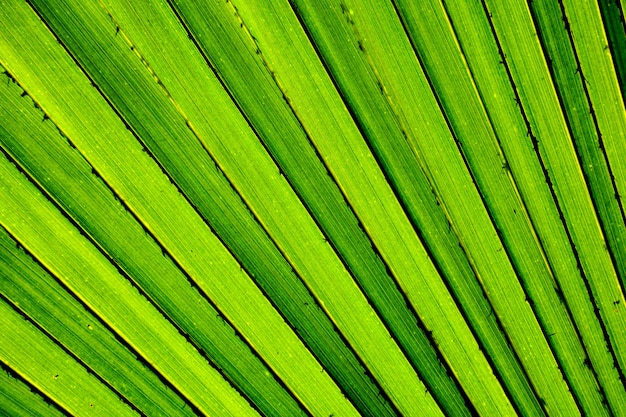This is a close-up photograph featuring a vivid green plant. The image showcases several stalks that might belong to bamboo or a similar plant, lined up in a row. The stalks are separated by thin, black lines, which could also be interpreted as shadows or gaps between the stems. The texture appears almost furry in places, adding to the organic feel of the photograph. The perspective is intriguing, leaving one to question whether they are viewing the plant through a microscope or possibly even an aerial shot of verdant fields and hedgerows. The green color dominates the image, giving it a fresh, lively appearance.